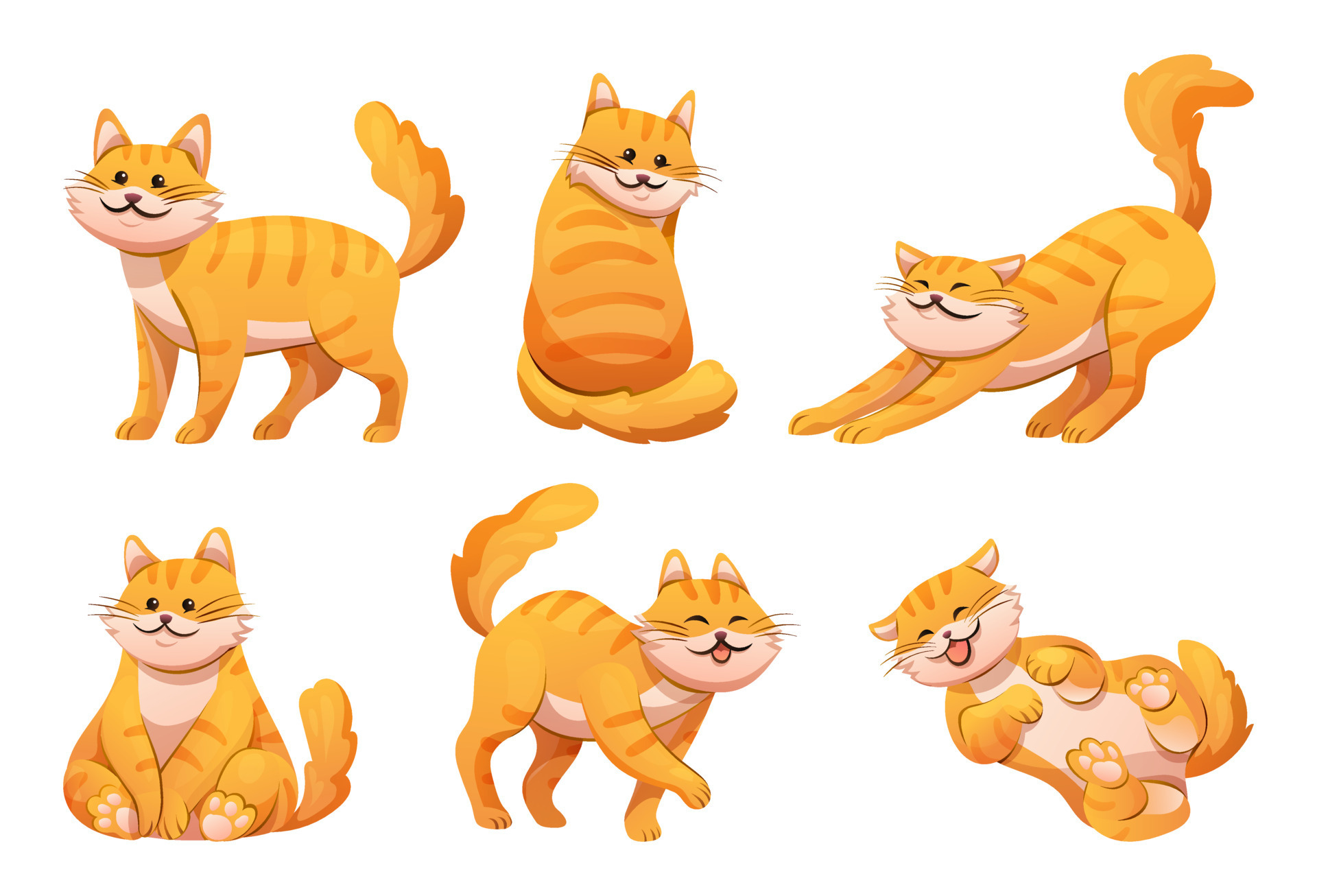This digital collage depicts a single orange cat with a white belly and dark orange stripes, captured in six distinct positions against a transparent background. In the top left image, the cat is seen standing on all fours, facing left, and smiling directly at the viewer. The second image shows the cat sitting with its back turned, head swiveled around to maintain its engaging smile. In the third position, the cat’s back is arched with its front legs stretched forward as if scratching the ground, eyes closed, embodying a playful stretch. The bottom left image portrays the cat sitting upright with its paws neatly placed in front, still smiling. In the fifth image, the cat is depicted mid-prance, further displaying its joyful personality. The final image in the bottom right corner shows the cat lying on its back, belly exposed, and tongue out, adding a touch of whimsy to its character. Each pose accentuates the cat’s cheerful demeanor, highlighted by its distinctive orange and white fur pattern.